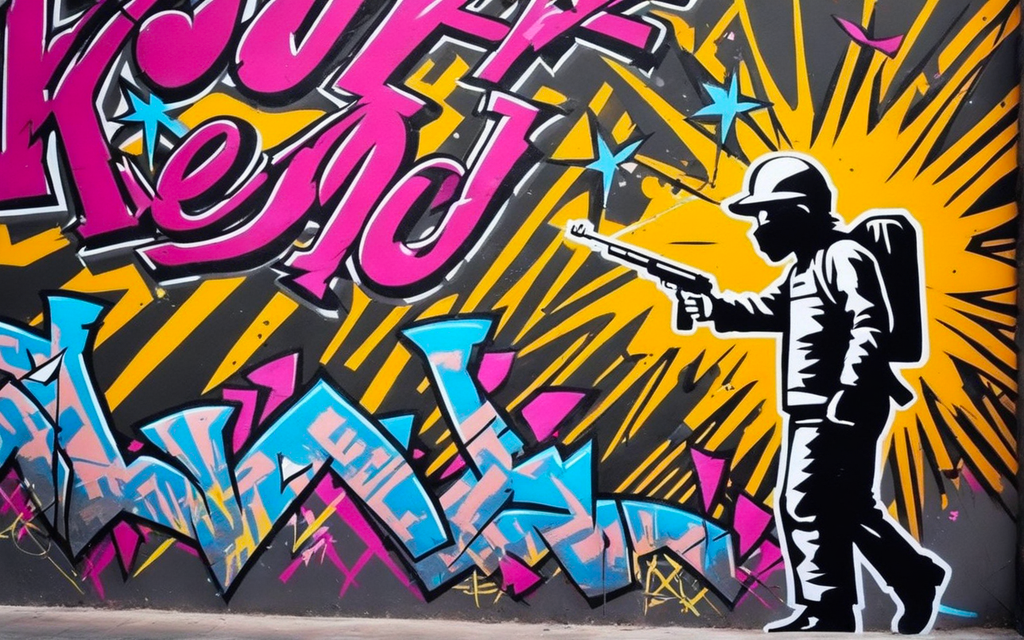The photograph captures a detailed mural painted on the side of a dark gray building. The central focus is a black and white figure of a man positioned towards the right, walking to the left. He is wearing a helmet, a mask covering the lower part of his face, a backpack, a sweatshirt, long pants, and boots. In his right hand, he holds a gun that resembles a pistol but with a rifle sight on it. Behind this figure, there is a dynamic yellow starburst explosion resembling a comic book "kapow," with orange cloud-like outlines. Large, pink, 3D graffiti-style lettering, partially readable with fragments of the letters "K," "E," and "J," is visible above and to the left of the figure. Additionally, there are blue stars scattered around, and more graffiti text stretches across the bottom in stylistic blue and white. The mural also features some pink triangular accents. The photograph includes part of a gray road or sidewalk at the bottom, anchoring the vibrant artwork against the urban backdrop.